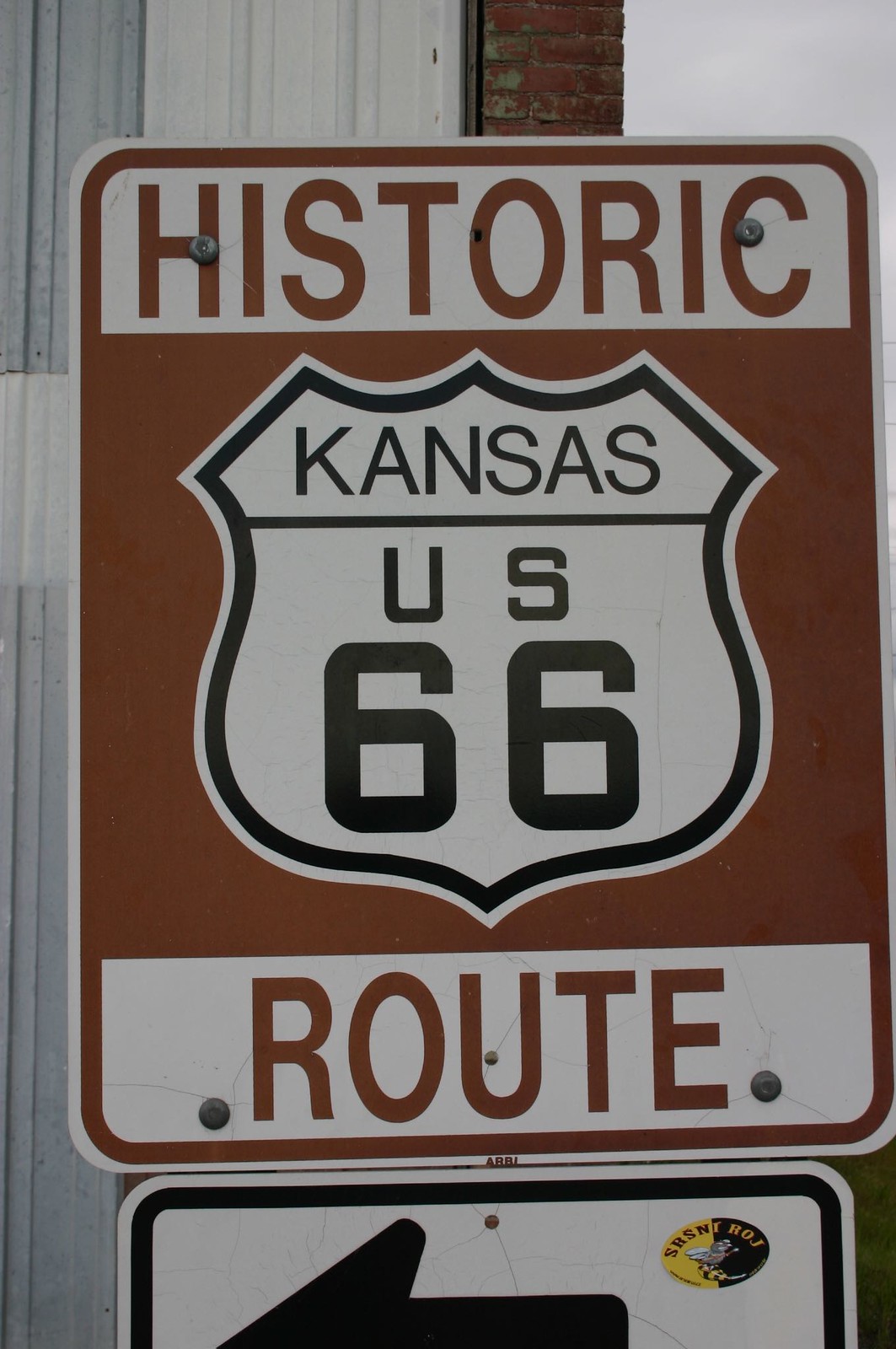This photograph showcases a historical road sign affixed to the side of a corrugated metal building with a hint of brick visible at the front. The primary sign, set against a white background, features a prominent red section with a white shield in the center. The shield displays the text "Kansas U.S. 66" in black letters. Above and below the red center are white rectangles; the top one reads "Historic" in red letters, and the bottom one reads "Route" similarly in red. Below this main sign, there is a partially visible secondary sign, also on a white background with a black border. This second sign includes a cropped black arrow pointing left and has a small yellow and black sticker in its upper right corner. The signs are clearly meant to guide travelers along the iconic U.S. Route 66 in Kansas.